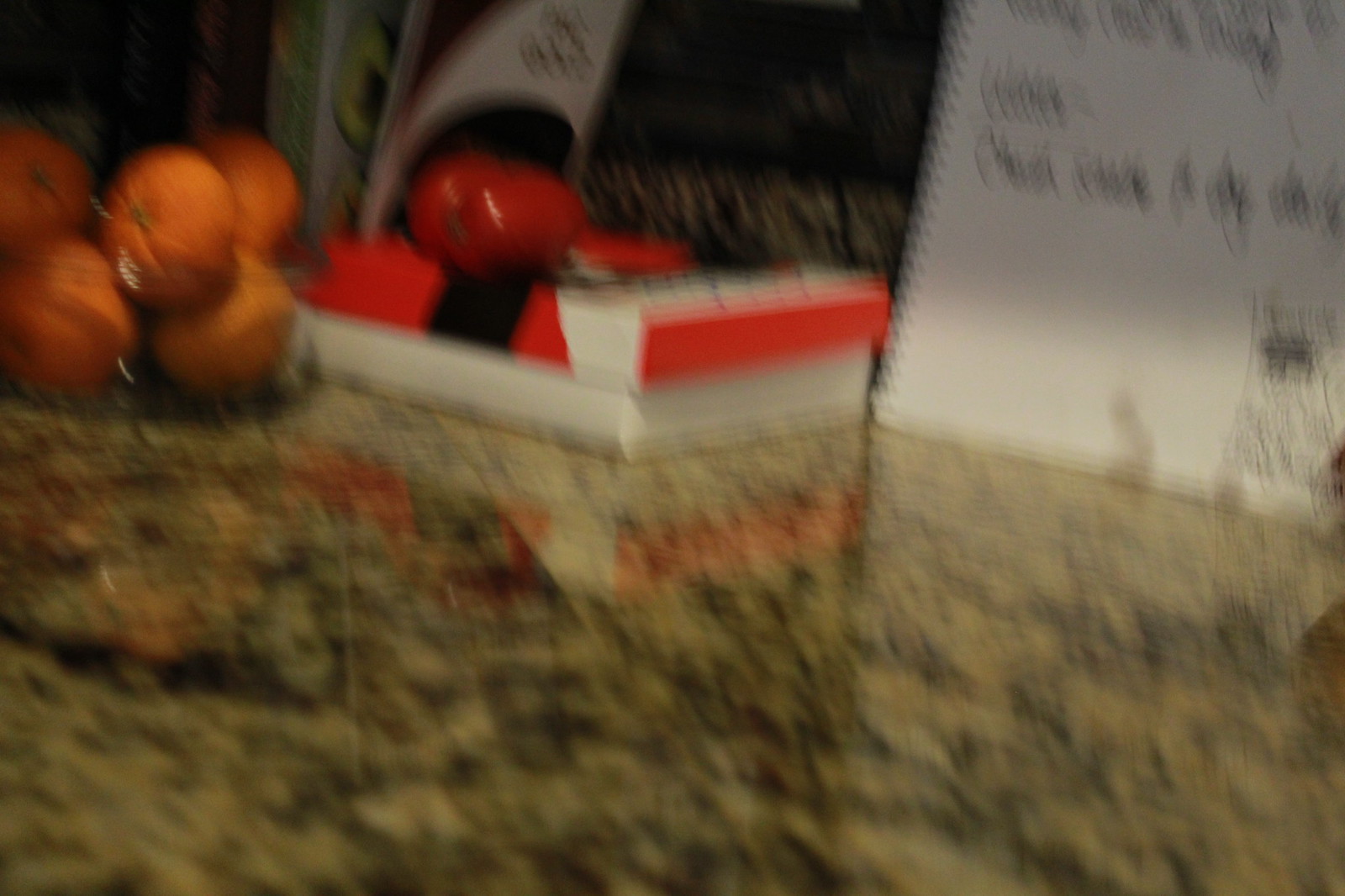The image depicts a blurry scene with objects placed on a surface that appears to be stone or marble. The surface, which is likely light brown or beige, features a marbled pattern in shades of yellow, brown, and darker hues, possibly black. The objects on the surface create a reflection, emphasizing the smoothness of the material. 

Among the items, there is a bag of oranges. Although the bag itself isn't distinctly visible, the arrangement of the oranges suggests they are contained within it. The oranges appear brownish due to the blur. Additionally, there is a box with a striking color scheme of red, black, and white. The box includes a depiction that resembles a small, red pepper. 

Behind these items, a loose-leaf binder or notebook is partially visible. The binder has white pages on the right side with black cursive writing—though the text is unreadable—and a black and white cover on the left. This collection of items is arranged at varying distances from the camera, contributing to the overall blurred effect of the photo.